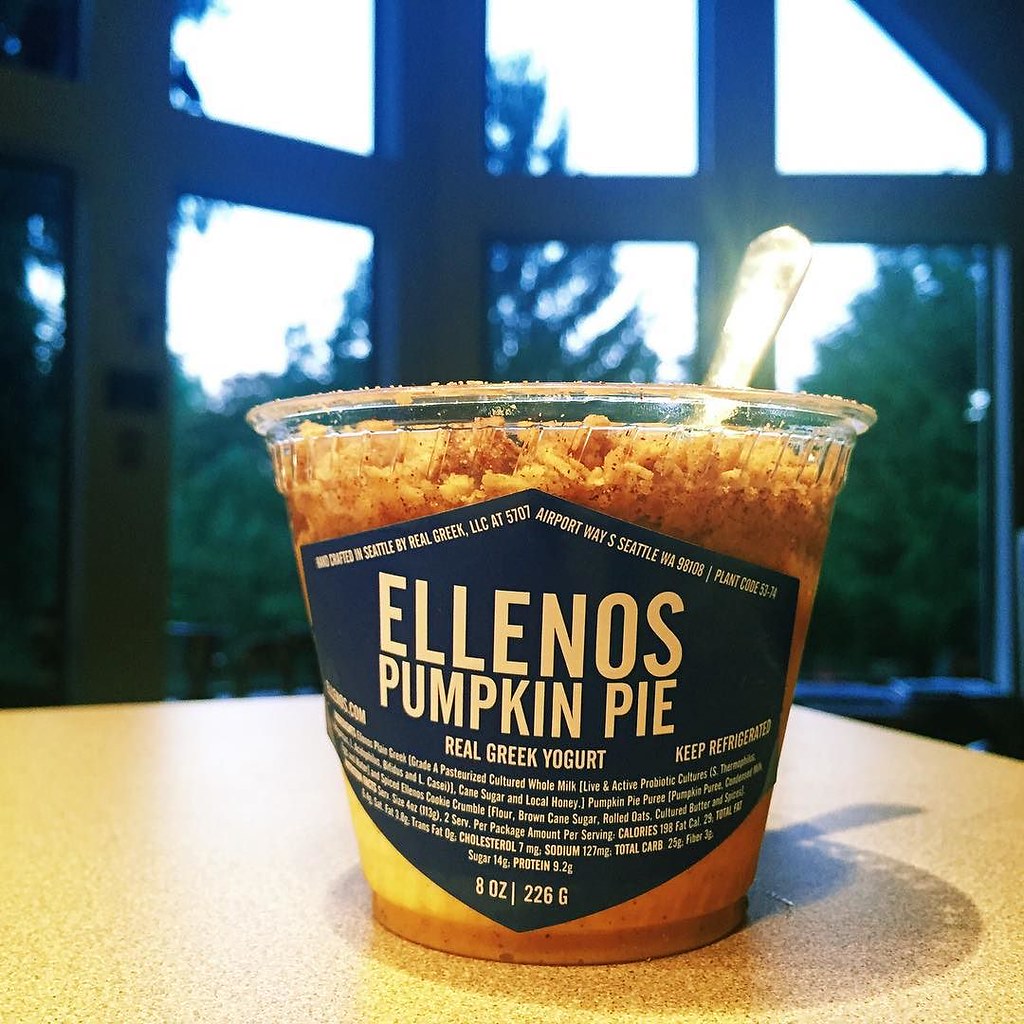The photograph captures a clear plastic cup containing Elleno's Pumpkin Pie Real Greek Yogurt, which is brown-orange in color with a creamy, slightly squishy texture. A silver spoon is inserted into the yogurt. The container is adorned with a distinctive dark blue shield-shaped label that prominently displays the text "Elleno's Pumpkin Pie Real Greek Yogurt" in bold white print. It also advises to "Keep Refrigerated" and provides details about its manufacture by Real Greek LLC, located at 5707 Airport Way, South Seattle, Washington, with a zip code of 98108. The net weight is indicated as 8 ounces or 226 grams.

The cup is positioned on a light tan stone countertop, casting a shadow on the surface. In the background, there is a large, floor-to-ceiling window divided into grid panes, through which blurry trees are visible, indicating it's daytime. The ingredients are listed on the label, though they are small and difficult to read. The overall setting suggests a serene indoor environment with natural light filtering through, partly illuminating the scene.